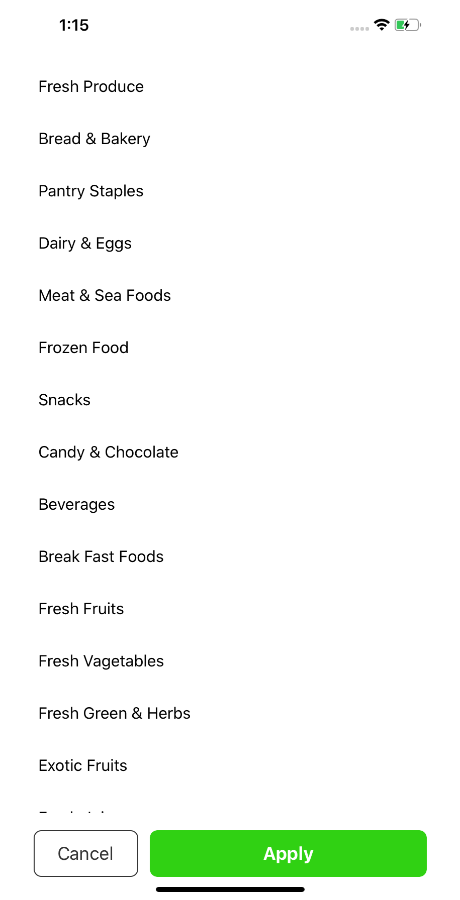The image is a vertically oriented screenshot against a black background, depicting a mobile app interface, presumably for grocery shopping. The phone display, set on a white background, reveals an app with an evident focus on grocery categories. At the top left corner, there is a numerical display, which ambiguously reads either "115" or "116." The top right corner of the image shows standard phone indicators, including a Wi-Fi symbol and a battery icon with only two green notches remaining.

A vertical list of grocery categories occupies the left side of the image. The distinct categories listed are: "Fresh Produce," "Bread and Bakery," "Pantry Staples," "Dairy and Eggs," "Meat and Seafood," "Frozen Foods," "Snacks, Candy, and Chocolate," "Beverages," "Breakfast Foods," "Fresh Fruits," "Fresh Vegetables," "Fresh Green and Herbs," and "Exotic Fruits." Although these categories are part of a longer list, only the tops of additional letters are visible above a "Cancel" button, indicating the list continues beyond the visible portion.

To the right of the "Cancel" button, there is a larger, rectangular button with a green background and the word "Apply" in white text. Beneath this interface, there is a long black dash, but no additional text or imagery is present beyond this point. 

Overall, the image succinctly captures the straightforward and categorized design of a grocery shopping app interface.